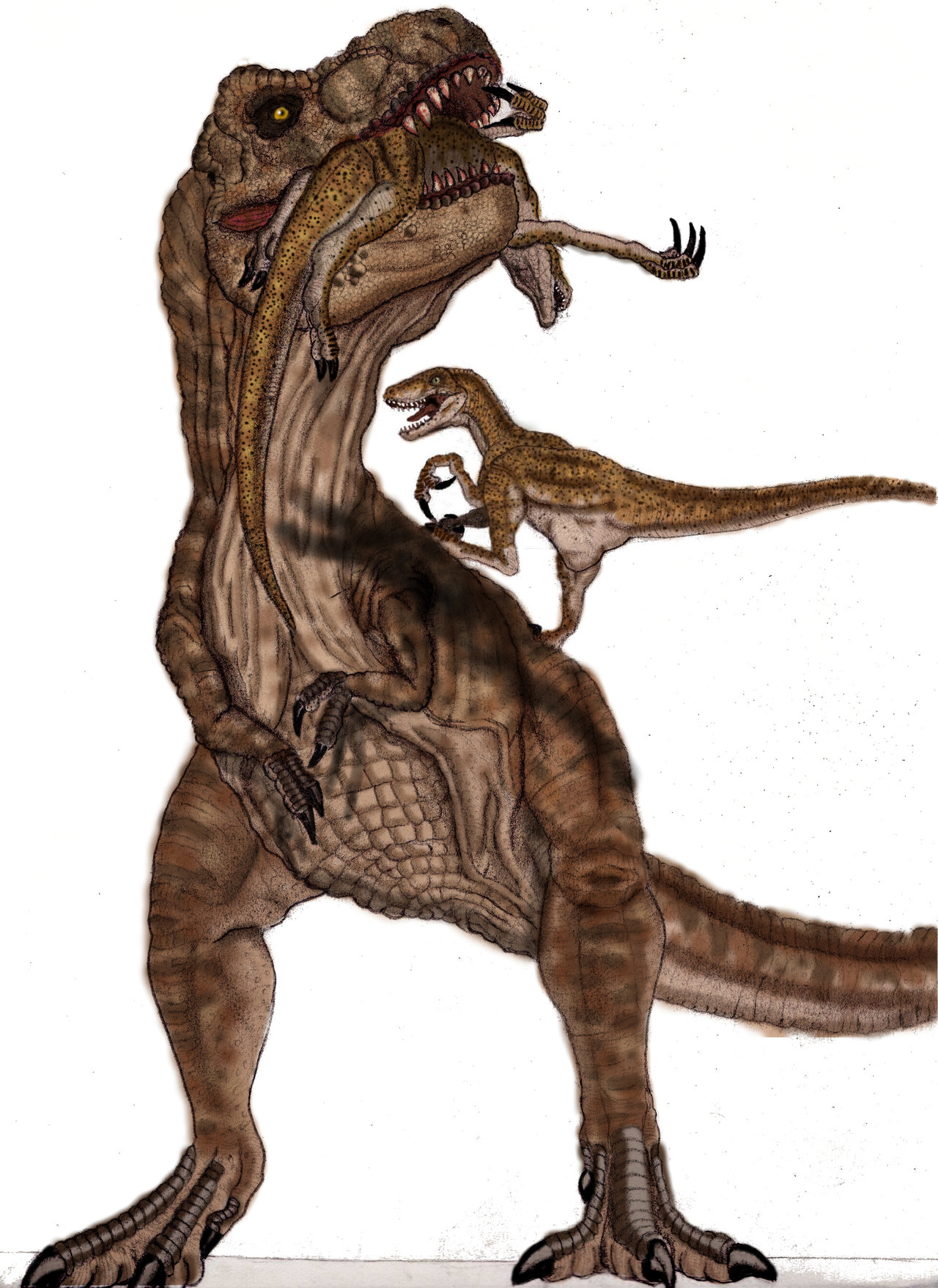This image appears to be a finely crafted piece of hand-made artwork depicting a detailed scene featuring several dinosaurs. The centerpiece is a ferocious Tyrannosaurus Rex, standing upright on a gray floor against a white background. The T-Rex, primarily colored in various shades of green with textured skin and scales, faces forward with its head turned slightly to the right. Its sizeable, menacing white teeth are sunk into a limp, green, black-spotted Velociraptor, which hangs lifelessly in the T-Rex's mouth, its tail draped and arms visible on either side. 

Another Velociraptor, also green but of a different hue, is perched on the T-Rex’s back, casting a long shadow on its side. This secondary Velociraptor has its mouth open, revealing sharp teeth, but appears to be merely climbing rather than attacking. The artwork reflects meticulous details such as a grid-like texture on the T-Rex's belly and large claws on its feet, indicating the use of possibly watercolor to achieve this effect. Overall, the scene conveys a sense of danger and raw power, capturing the intense, predatory nature of these prehistoric creatures.